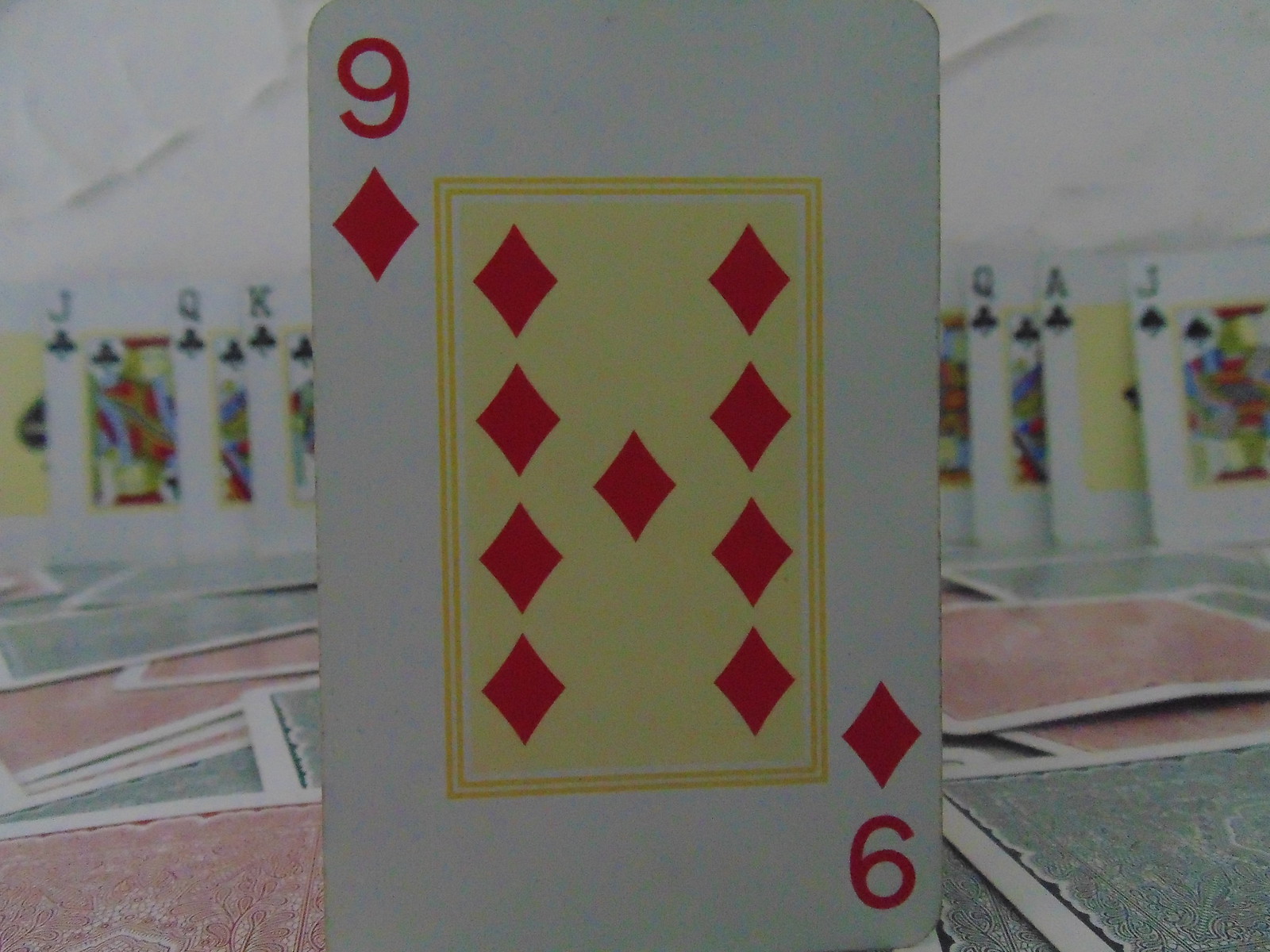In this dimly lit photograph, the focus is on a vintage deck of playing cards, with the nine of diamonds prominently displayed in the foreground. The card design is simple, featuring a standardized number "9" and an arrangement of nine red diamonds in an H pattern set within a subtle yellow rectangle. The surrounding cards include the Jack of Clubs, Queen of Clubs, King of Clubs, and various spades, all miniaturized to about one-third the size of the nine of diamonds, adding depth to the scene. In the background, another set of cards lies face-down, exhibiting signs of wear and slight bends, indicating they have been used frequently. The backdrop features a light gray, textured wall with visible ridges, suggesting a hasty plastering or painting job, contributing to the overall vintage and somewhat worn aesthetic of the image.